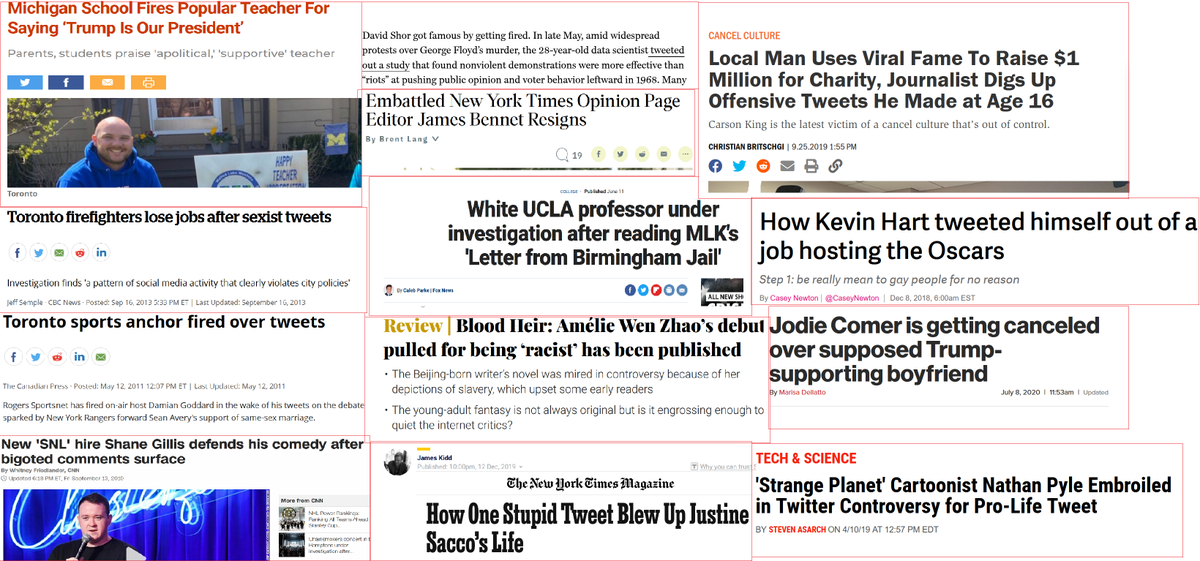The image depicts a collage of controversial headlines, each enclosed within a red border, arranged in three columns. The top-left headline reads, "Michigan School Fires Popular Teacher for Saying Trump is Our President," printed in red font. Adjacent to it is a picture of a man in a blue hoodie smiling. Below it, another headline states, "Toronto Firefighter Loses Job After Sexist Tweets," followed by "Toronto Sports Anchor Fired Over Tweets." At the bottom of the left column, "New SNL Hire Shane Gillis Defends His Comedy After Bigoted Comments Surfaced" is displayed, featuring a photo of a white man in front of a blue curtain giving a comedy talk.

The central column begins with a headline about David Shore: "David Shore Got Famous by Getting Fired in Late May Amid Widespread Protests Over George Floyd’s Murder." This is followed by "Embattled New York Times Opinion Page Editor James Bennett Resigns." Further down, "White UCLA Professor Under Investigation After Reading ML King’s Letter from Birmingham Jail" is featured, then "Review: Blood Air, Emily Nguyen-Zho’s Debut Pulled from Being Racist Has Been Published." The column concludes with "How One Stupid Tweet Blew Up Justin Seto’s Life," accompanied by social media icons like Facebook, Twitter, and LinkedIn, suggesting the headlines could be shared on these platforms.

In the right column, the top headline is tagged with an orange "Cancel Culture" label and reads, "Local Man Uses Viral Fame to Raise One Million for Charity; Journalist Digs Up Offensive Tweet He Made at Age 16." Below it, "How Kevin Hart Tweeted Himself Out of a Job Hosting Oscars" is highlighted, summarizing with "Step One, Be Really Mean to Gay People for No Reason." Another headline states, "Jody Comer is Eating Cancel Over Supposedly Supporting Boyfriend." Finally, the column ends with "Tech and Science: Strange Planet Cartoonist Nathan Pyle Embroiled in Twitter Controversy for Pro-Life Tweet."

The entire assembly of headlines, numbering twelve in total, is visually arranged into three balanced columns, conveying a tapestry of publicized controversies encapsulated in small, red-bordered boxes.